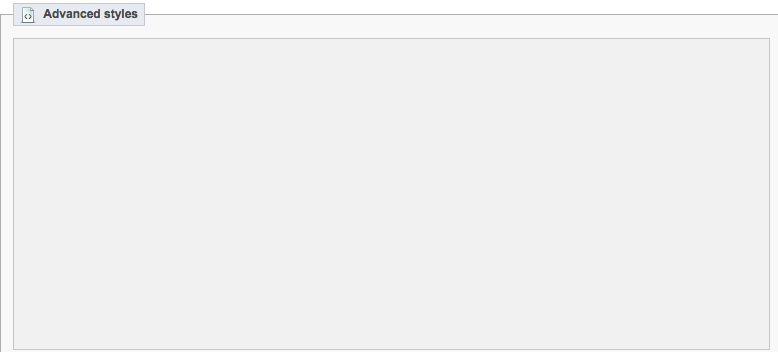The image features a plain, elongated gray box set against a neutral background. Encircling the gray box is a thin line, lending it definition. Positioned at the upper left corner of the box is the phrase "Advanced Styles," written in black with a subtle gray shadow effect. Adjacent to this text is an icon resembling a white piece of paper with an undecipherable symbol at its center. The elements and layout suggest a user interface component, possibly related to advanced styling options within a computer system or software application.